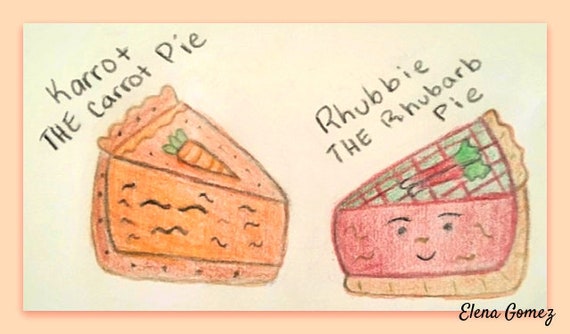The image showcases a hand-drawn picture, likely created by a child, of two slices of pie framed as a painting with a light orange border. On the left side is a detailed drawing of a carrot cake with an orange crust and filling, labeled as "Karrot, the carrot pie." The right side features a slice of rhubarb pie, called "Ruby, the rhubarb pie," which is red with a brown crust and includes a rhubarb piece on top, plus a smiley face on its side. The drawings are colored with crayon, giving them a vibrant, textured look. The artist's name, Elena Gomez, is clearly written at the bottom of the image, which is set against a white background laid over a pink one.